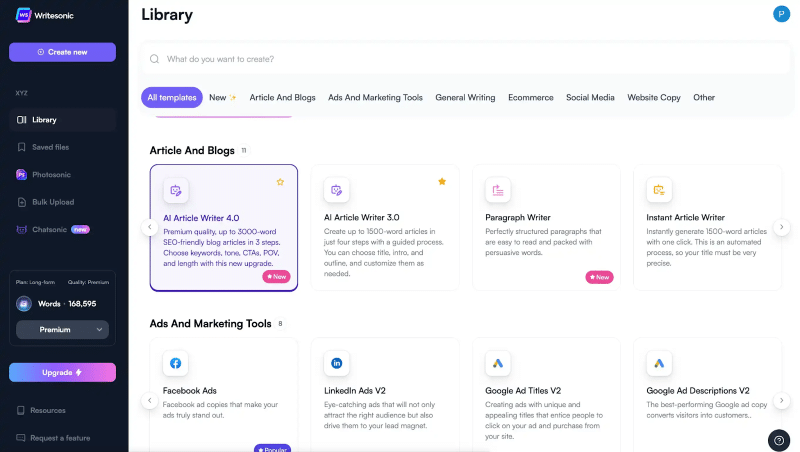Detailed Caption:

The image depicts a comprehensive user interface for a writing and content creation platform. In the top left corner, the interface displays the "Write Sonic" logo followed by an option labeled "Create New." Below this, there is a series of menu items including "XYZ," "Library," "Save Files," "Photosonic," "Bulk Upload," "Chat Sonic," and a label reading "New."

Adjacent to these, the interface features additional options categorized under "Plan," which include subcategories such as "Long Term," "Quality," "Premium," and "Words." Options to "Save" work are visible. The interface also provides a drop-down menu for "Premium," with additional selections for "Upgrade," "Resources," and "Request a Feature."

Below the top menu is another row containing categories like "All Templates," "New," "Article and Blogs," "Ads and Marketing Tools," "General Writing," "E-commerce," "Social Media," "Website Copy," and "Other." Specifically highlighted are "Article and Blogs" and "Article Writer 4.0" which comes with "Premium Quality" and allows for creating up to 3000-word SEO-friendly articles. Additional features include options for "Keywords," "Tones," "CTAs," and "POV."

The interface also mentions "Article Writer 3.0," which offers a guided process to create up to 1500-word articles in four steps: selecting a Title, Intro, Outline, and Custom Fonts. The platform promises perfectly structured paragraphs that are easy to read and can generate 1500-word articles instantly through this automated process.

In the top right corner of the interface, there is a blue circle with a "P" in the middle, possibly representing profile or premium status. The overall layout is designed to facilitate various content creation needs through an organized and user-friendly interface.